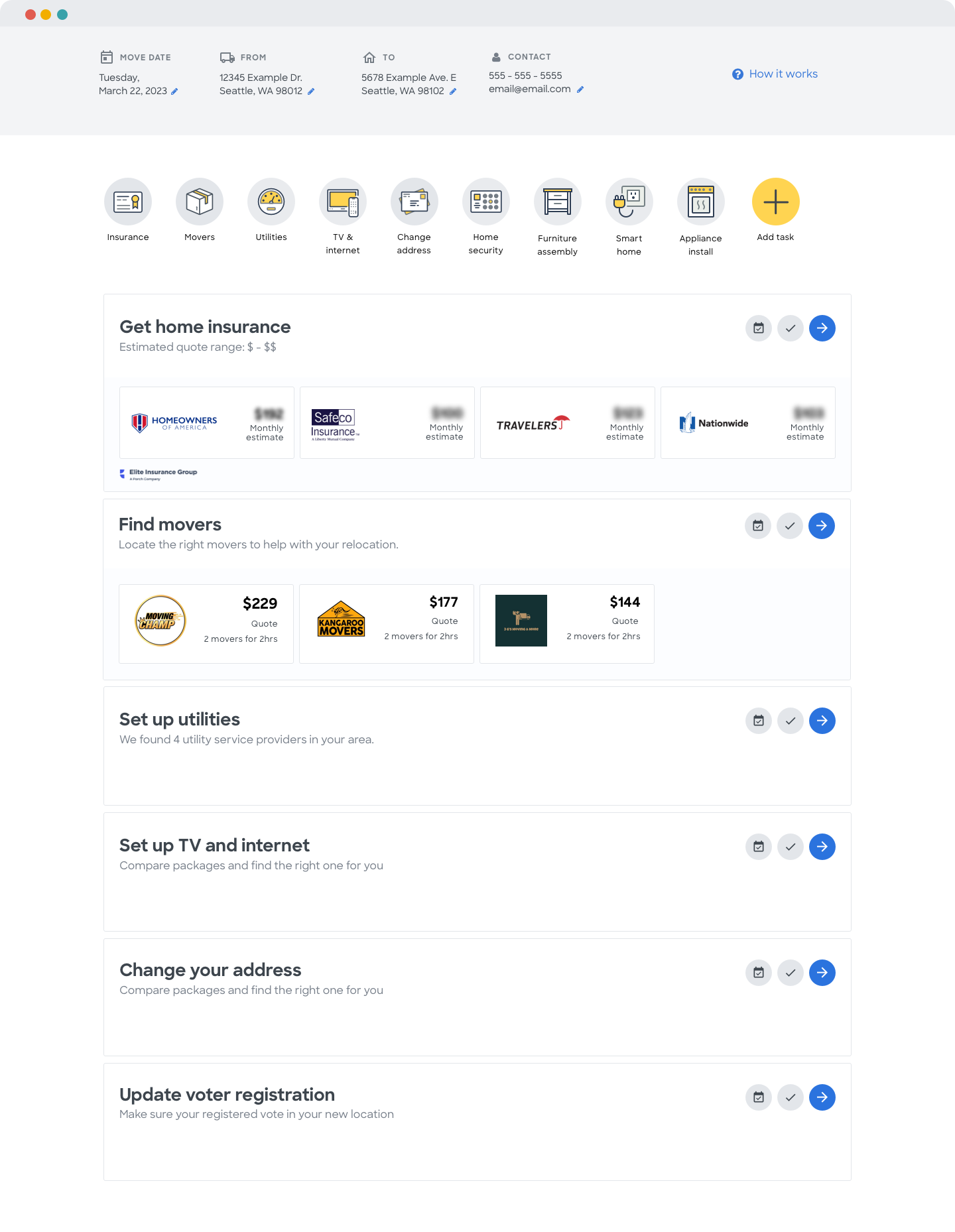The image depicts a software interface, likely from a program on an Apple computer or tablet, designed to assist individuals who have recently purchased a new house and are planning their move. The interface features a gray header at the top displaying information fields for the move date, the address being moved from, and the destination address, indicating that it could also be coordinating with a moving company.

Below the header, the interface displays a series of icons representing various aspects of the moving process including: 

- Insurance
- Movers
- Utilities
- TV and Internet
- Change of Address
- Home Security
- Furniture Assembly
- Smart Home Setup
- Appliance Installation
- An option to add additional items

These icons are also listed in a detailed format beneath the icon row, each with a corresponding action button. For each task, users can plan, schedule via a calendar feature, and mark tasks as completed. Each item in the list has an arrow that likely allows the user to access further options or perform specific actions related to the task.

The first item in the list is "Get Home Insurance," displaying logos of various insurance companies for easy selection. Directly below this is "Find Movers," which shows quotes from different moving companies. Other categories continue further down, providing a comprehensive set of tools to manage the entire moving process efficiently.